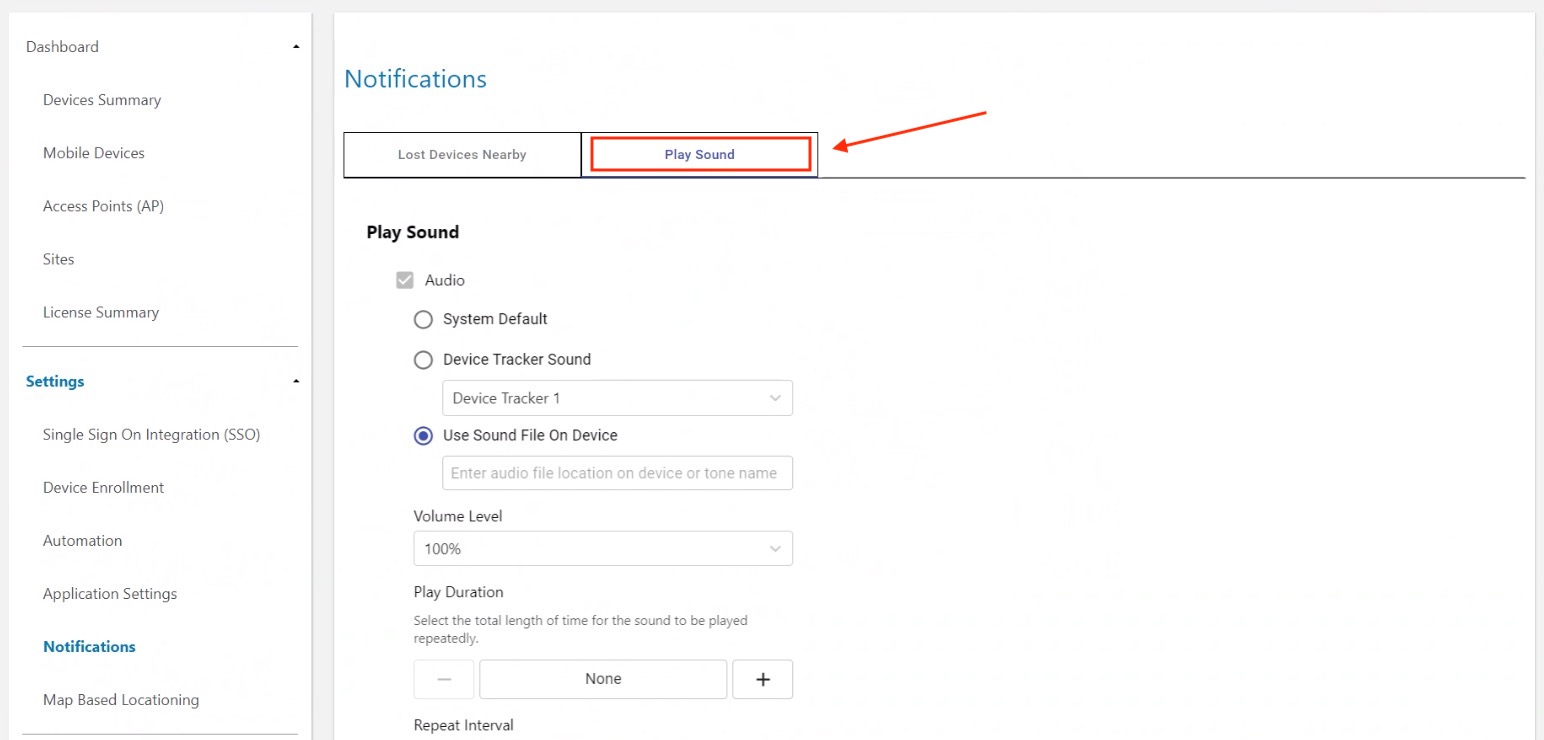The image depicts a comprehensive dashboard interface, primarily divided into a left pane and a main content area. The left pane lists various options, including "Devices Summary," "Mobile Devices," "Access Points," "Sites," "License Summary," "More Settings," "Single Sign-On Integration (SSO)," "Device Enrollment," "Automation," "Application Settings," and "Map-Based Locationing." 

In this particular scenario, one of the options, "Notifications," has been selected, bringing up the corresponding page in the main content area. This page is focused on features related to lost devices, including sections like "Lost," "Devices Nearby," and "Play Sound." 

Highlighted within this page is the "Play Sound" button, indicated by an arrow pointing towards it. This functionality appears to be intended for locating a lost device, possibly a phone, which is linked to the system. By clicking the "Play Sound" button, the user can trigger a sound on the lost device, assuming the device is correctly integrated with the system.

The user has multiple customization options for the sound to be played. They can choose between "System Default," "Device Tracker Sound," or "Use Sound File on Device." If choosing the latter, they can specify the file path for the sound file. Additional settings allow adjustments to the volume level, with a current setting of 100%, the duration the sound will play, and the repeating intervals. These options provide flexibility in ensuring the sound is both noticeable and appropriate for the situation.